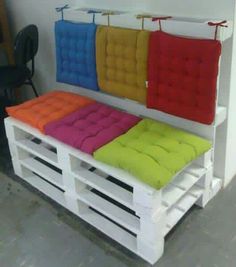In this image, there is a unique modular seating area constructed with a white, crate-like stacking system. The structure can be adjusted to various heights, starting close to the floor and stacking up to the height of a regular chair, with small leg sections about six inches high. The seating unit also features a backrest made by stacking additional modular pieces. Brightly colored cushions are both hanging from the upright backrest and lying on top of the stacked seating elements, giving it the appearance of a vibrant couch. The cushions are in varied hues including orange, red, green, blue, brown, maroon, magenta pink, purple/violet, and a muted yellow. Hanging cushions are secured with visible bow-tied strings. This adaptable setup hints at a possible inspiration from Japanese-style floor seating, allowing the seating to transform from a floor-level arrangement to a higher, more conventional couch-like configuration.